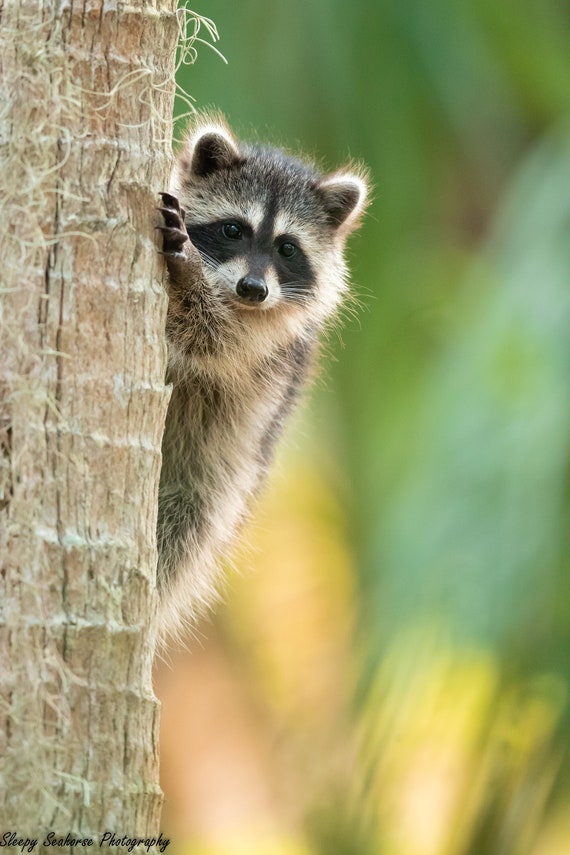The image captures a young raccoon peeking from behind a tree trunk or wooden post in a bright, daytime setting. The raccoon is climbing the wood, which has small white fibers on it. Its left paw with sharp, dark claws is visible. The raccoon’s fur is a mix of gray, brown, beige, black, and white. It has distinctive black and white facial markings, with shiny black beady eyes and a black nose. The background is a muted blur of green and yellow, suggesting trees or leaves. In the bottom left corner, there is a watermark crediting Sleepy Seahorse Photography.